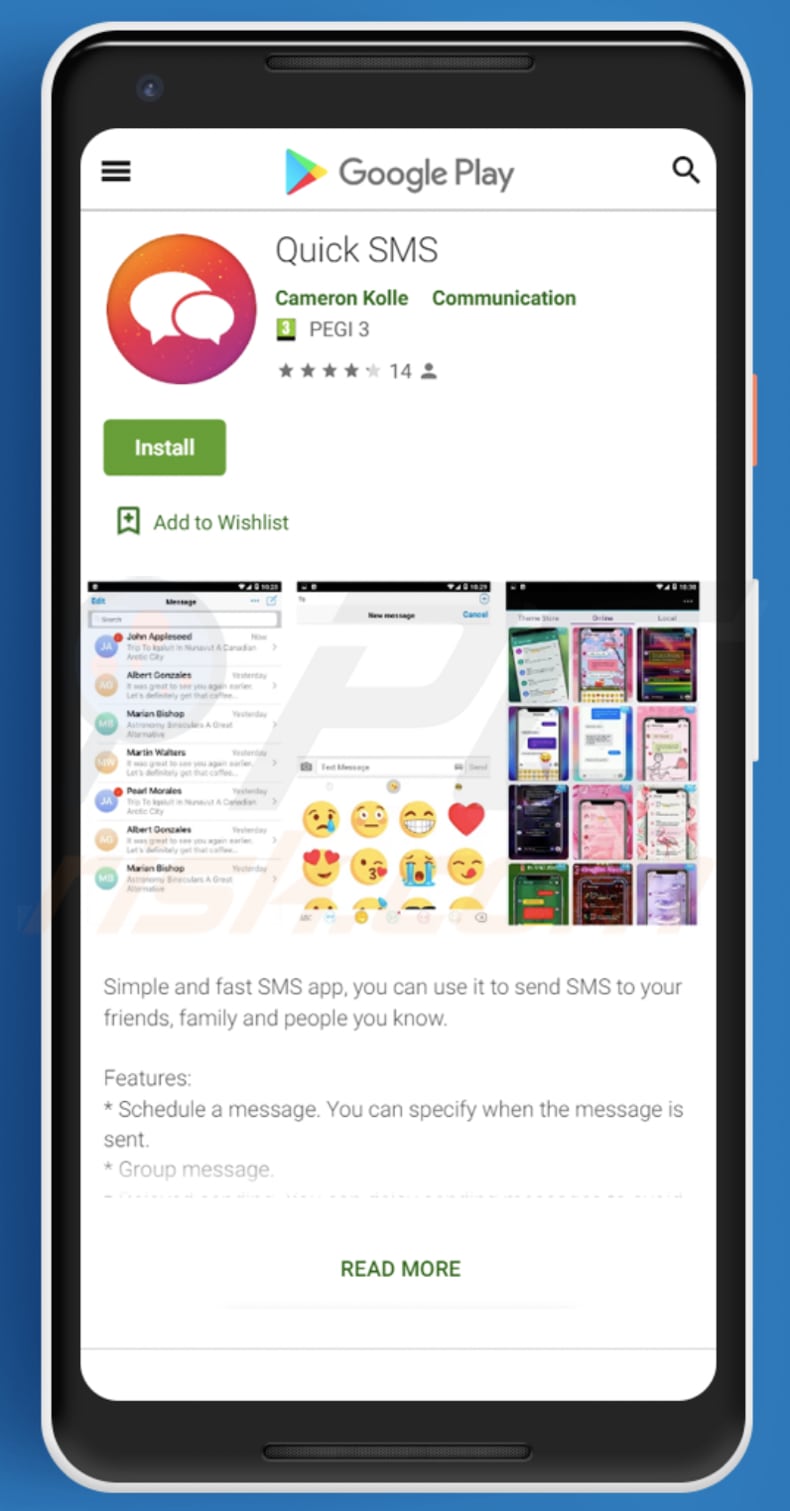The image captures the front view of a smartphone screen displaying the Google Play Store interface. Positioned at the top left is the front-facing camera, directly next to the centrally-located speaker. The bottom edge houses the microphone. The active screen shows the Google Play Store with a search icon on the right and a menu icon on the left. Below these icons, an app is prominently featured: "Quick SMS" identified by a circular logo with two chat bubbles inside.

Key details of the app are also visible:
- Name: Quick SMS
- Category: Communication
- Developer: Listed below the app name
- Rating: 4 out of 5 stars, based on 14 reviews
- Install Button: A green "Install" button is present below the app logo.

Additional elements include:
- Wishlist: A bookmark icon labeled "Add to Wishlist"
- Preview Images: Three still shots showcasing the app's features such as different backgrounds, emojis, and chat formats.
- Description: The text underneath summarizes the app as a "Simple and fast SMS app" for sending messages to friends, family, and acquaintances.
- Features: Lists functionalities like message scheduling and group messaging.
- Further Information: The last portion of the description fades out, indicating more content which can be revealed by scrolling. A "READ MORE" prompt in capital letters hints at additional details but is non-clickable.

Below the descriptive text is a glimpse of grayed-out information, suggesting that further scrolling would reveal more about the app.